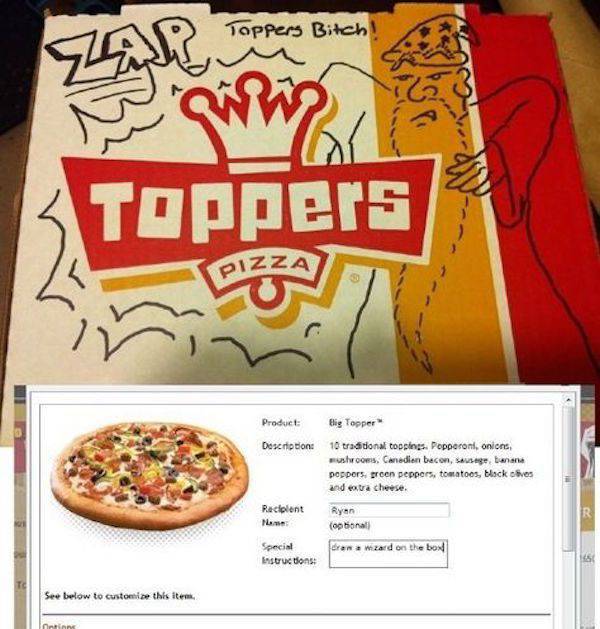In this image, there is a large closed pizza box positioned towards the top against an indistinguishable background. The box prominently features the logo "Topper's Pizza," with "Topper's" displayed in a jumbled, toppled-over font, partially obscured by a white crown with a red outline and a gold shadow. Below, the word "Pizza" is clearly visible in bold. On the right-hand side of the box, there is a hand-drawn wizard in black marker with a long beard and a starry hat, saying "Topper's Bitch!" The word "Zap" appears in the top right corner.

The box, decorated in colors of tan, black, red, orange, green, and white, includes a detailed description of the pizza order: "Big Topper" with ten traditional toppings—pepperoni, onions, mushrooms, Canadian bacon, sausage, banana peppers, green peppers, tomatoes, black olives, and extra cheese. At the bottom, there's a screenshot from the website showing the order details. The recipient's name is Ryan, with special instructions to draw a wizard on the box. The setting appears to be inside someone's home, with the screenshot clearly indicating that the image is a digital upload, capturing both the pizza box and the order details from the website.